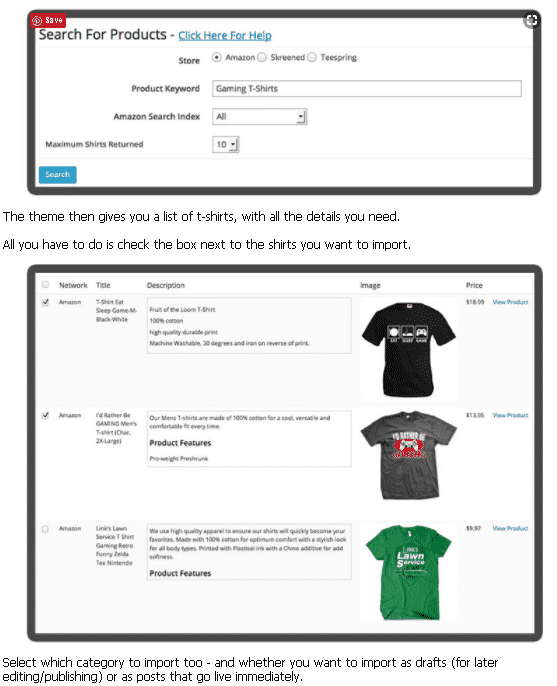**Detailed Caption:**

The vertically-oriented image displays a detailed instructional guide for a website or app that facilitates product searches and imports. 

**Top Section:**
The first screenshot at the top features a colorful interface where users can search for products. It presents options to seek help and allows the selection of various online stores such as Amazon, Screened, and Teespring. The keyword "gaming t-shirts" is typed into the search bar. The user has selected Amazon as the store and specified a maximum of 10 shirts to be returned by the search. Beneath this, a 'Search' button is available for initiating the query.

The description under the first screenshot explains that the theme provides a list of t-shirts with comprehensive details. It instructs users to check the boxes next to the desired shirts to import them.

**Bottom Section:**
The second screenshot beneath displays the search results for "gaming t-shirts" from Amazon. Each entry includes the title and price of the t-shirts. Examples of the top three results include:
1. "T-Shirt Sleep Game in Black and White" - $18.
2. "I'd Rather Be Gaming Men's T-Shirt" - $13.
3. "Lynx Lawn Service T-Shirt" - $9.
 
On the right side of each result, there is an option to "View Product" for more details and to save the item.

The image serves as a step-by-step guide, illustrating the interface and process of searching and selecting gaming t-shirts from Amazon using the software.